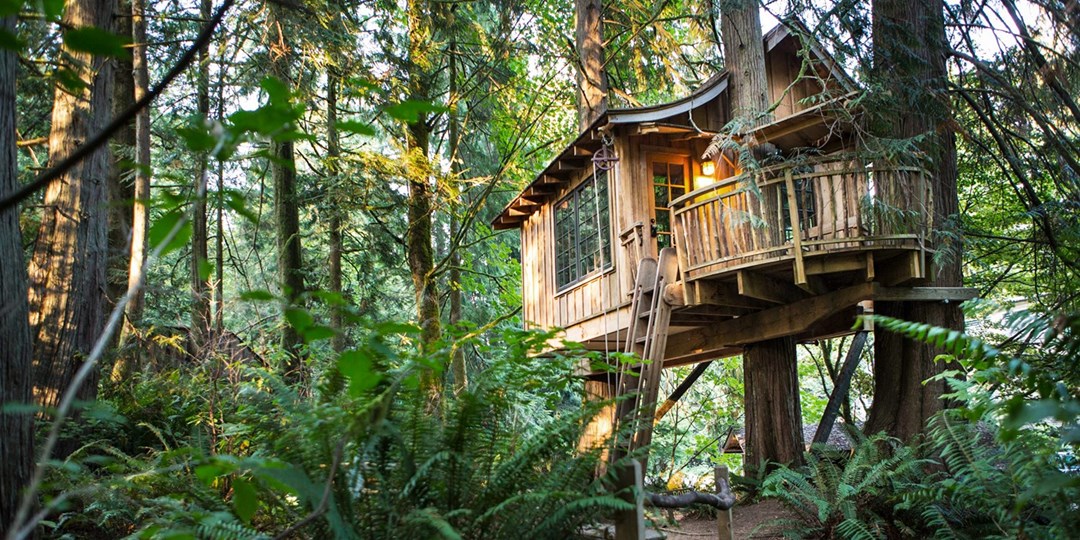In the midst of a densely wooded forest, a strikingly elegant and modern treehouse stands nestled among two large trees on the right. The backdrop is a rich tapestry of green leaves, tree trunks, and the clear blue sky peeking through the canopy. The ground is blanketed with low-level green plant life and ferns, adding to the serene woodland charm. The treehouse itself is a marvel—constructed from light brown wood with gray trim, featuring a sharply inclined pitched roof. Accessed by a gray wooden ladder leading to a charming half-circle balcony, the treehouse includes a wooden French door adorned with six glass panels, flanked by an orange glowing light. The side of the treehouse showcases an expansive picture window, beneath which the rafters extend out under the roof's edge. This cozy elevated abode, potentially an Airbnb retreat, invites visitors to experience a peaceful life amongst the trees.